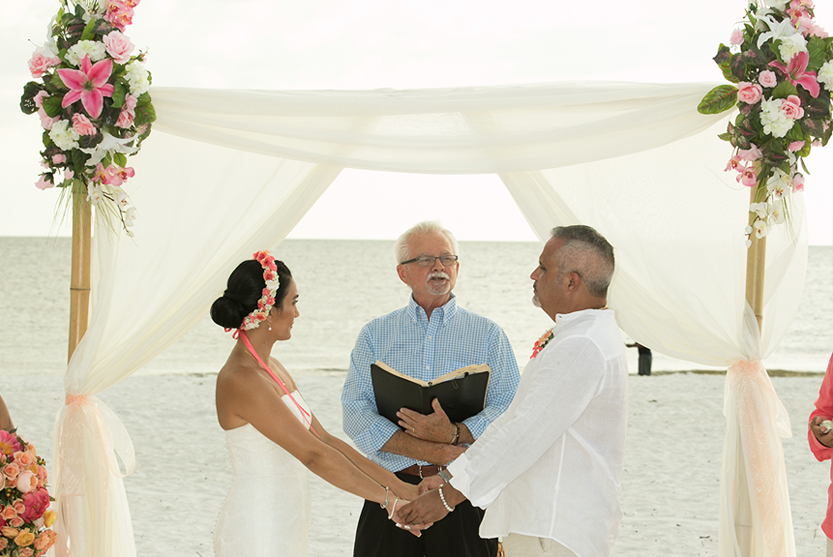In the image of a beach wedding, the couple stands on pristine white sands, holding hands and looking intently at the officiant ahead. The officiant, an older gentleman with a white beard, mustache, and short white hair, is adorned in glasses and a blue checkered shirt. He holds an open book, presumably containing the wedding vows. 

The bride, with an elegant updo and a flower crown of peach and white blooms, is dressed in a sleek, strapless white wedding gown. She stands opposite the groom, who is wearing a loose, white long-sleeve button-up shirt and tan or cream-colored pants. Around his neck is a flower necklace. 

They are both under a beautifully draped white cloth banner, adorned with florals, adding to the romantic ambiance of the beach setting. In the background, the serene ocean can be seen, enhancing the picturesque quality of this seaside wedding ceremony.